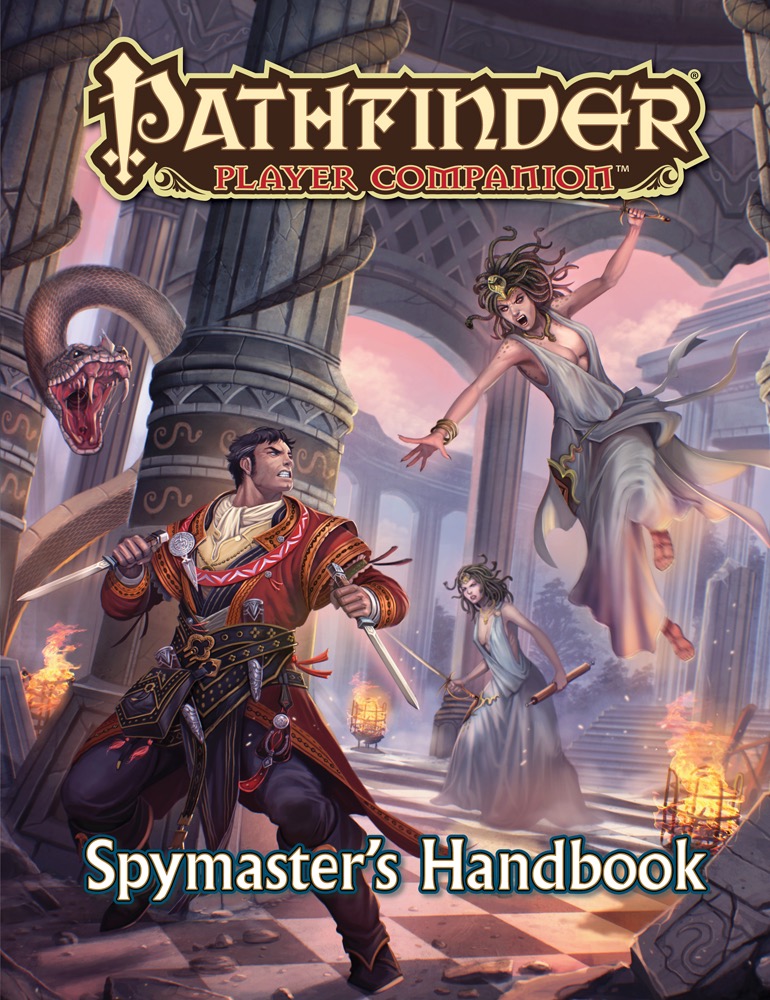This image is a digital book cover for the RPG-themed "Pathfinder Player Companion: Spymaster's Handbook." At the top, "Pathfinder Player Companion" is prominently displayed in a rustic, fantasy-style logo where the upright of the 'P' is cleverly designed as a sword pointing upwards. At the bottom, the title "Spymaster's Handbook" appears in a more standard white font. The scene depicts a dramatic confrontation set against a backdrop of Greek-inspired architecture, featuring marble columns, a checkered black-and-white floor, and lit fire sconces.

In the midst of the action, a swashbuckling hero dressed in a red coat, black pants, and a white corvette around his neck wields twin short swords, more akin to long blades than knives. He faces a range of threats: a large snake with menacing fangs and tentacle-like appendages wrapped around nearby pillars, and two Medusas—one observing from the background and another leaping through the air, seemingly poised for attack with her disheveled hair. The sky is tinged pink behind the temple-like setting, tying together the fantastical and perilous atmosphere.